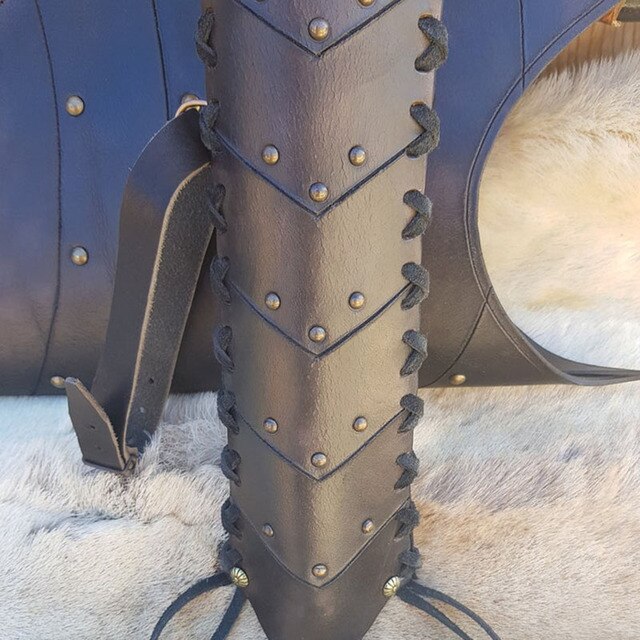The image appears to be a detailed photograph of a leather strap, likely part of a piece of tack commonly used on animals, such as a horse halter. The strap, made of brown leather, features sections joined by metallic rivets and decorated with gray shoelaces threaded through holes along the sides. The scene also shows a buckle on the left side of the strap, suggesting its purpose for tightening or securing something. The background consists of white, fluffy fur, further indicating that the strap is attached to an animal. The zoomed-in nature of the photograph makes it challenging to discern the complete item, but the combination of leather, rivets, and fur suggests an equestrian accessory designed for both function and stability.